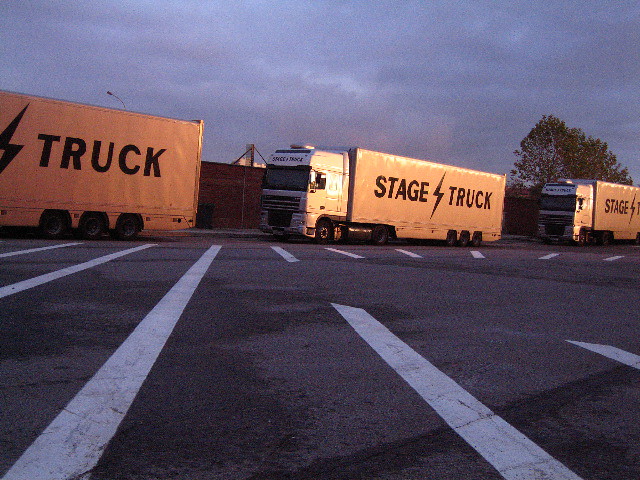This photograph depicts a parking lot where three large 18-wheeler trucks are parked in front of a wall, possibly made of brick. The trucks, which are prominently featured with "Stage Truck" written in black on their sides accompanied by a small lightning bolt between the words, have white cabs and either white or beige cargo sections. The image shows the side profiles of the trucks, with the middle truck being in full view. The parking lot surface has visible white lines and wet patches suggestive of recent rain. In the background, the sky is overcast with gray clouds, and several trees are visible to the right of the trucks. The overall clarity of the picture isn't the sharpest, giving it a somewhat muted appearance.